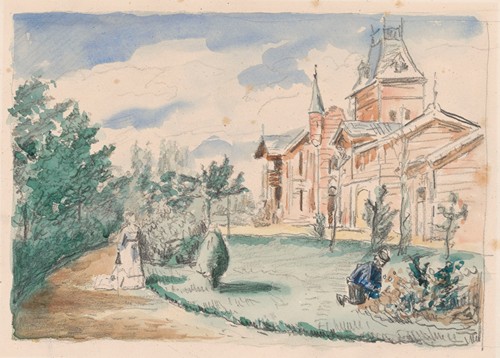The image depicts a delicate watercolor scene framed by a buff paper border of about one inch. Rendered in soft, unsaturated hues, the scene captures a serene moment in a garden. On the right side, a man, possibly of Chinese descent given his traditional attire, kneels attentively beside a small garden. Behind him, a sprawling red brick house with numerous towers, spires, and a weather vane rises impressively. This house features a complex architecture with varying roof heights, chimneys, and a balcony, giving the impression of a grand, multi-sectioned estate.

On the left, a circular driveway curves past manicured lawns and a tan walkway, leading up to the house. Trees are strategically placed around the scene, adding to the well-tended look of the garden. The sky above is painted in varying shades of blue with white clouds that appear to be sketched with faint pencil or pen strokes, enhancing the overall tranquility of the image. Amidst this picturesque setting, a woman in a white flowing Victorian gown strolls with a parasol in her hand, adding a sense of period charm to the scene.